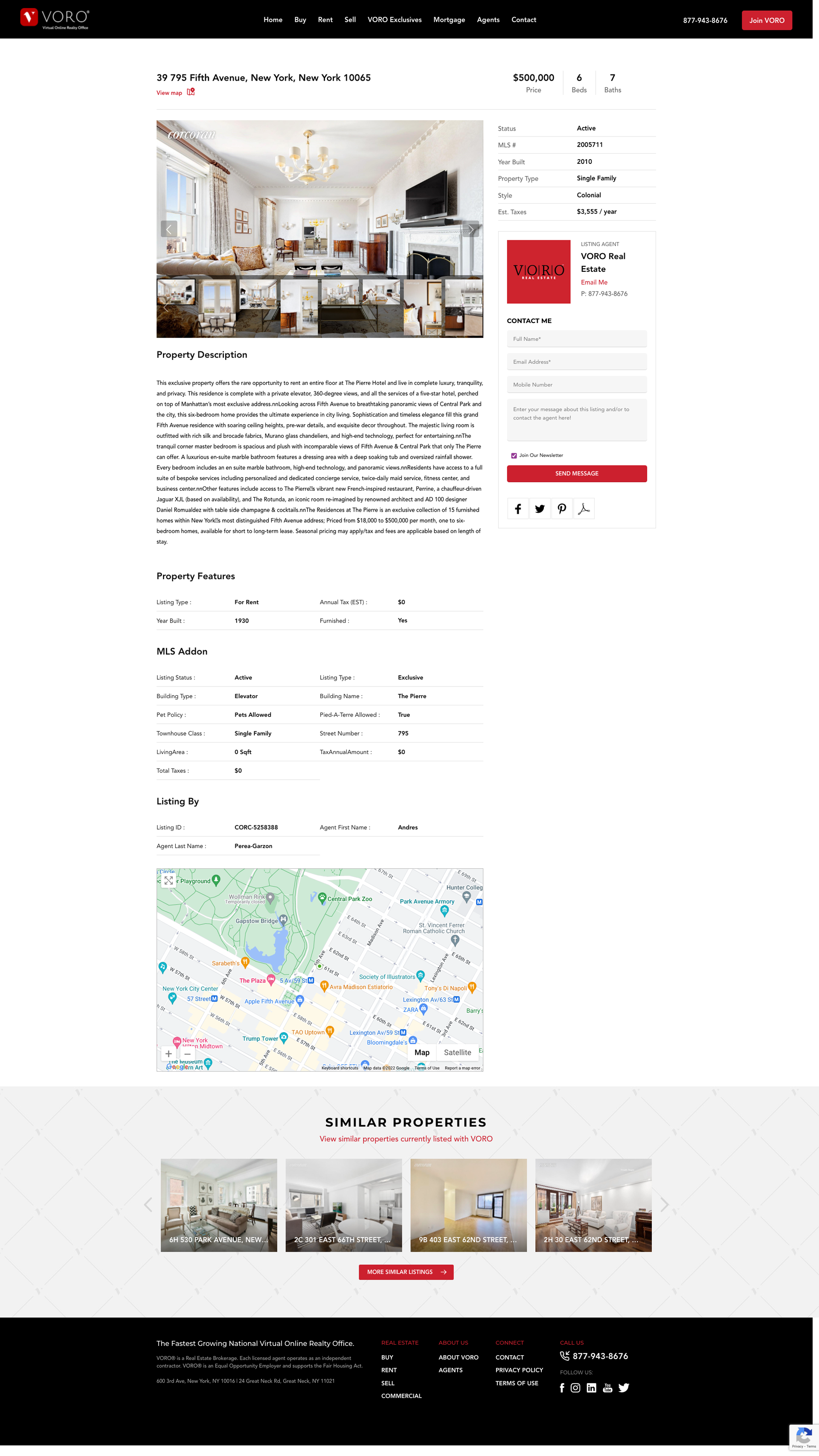The image displays a detailed real estate listing page with a white background. A prominent black bar divides the top section, underneath which is a photograph showcasing the interior of a house. A red square labeled "VRL" or possibly "vovo" is visible. Accompanying this are white words that are somewhat unclear, possibly reading "Property Description." 

The section below the photograph contains more detailed information, potentially about the property, including key details such as location and listing information. A red rectangle highlights critical data, perhaps property attributes or a price indicator. There is also a map feature with a couple of location icons pinpointing the property’s whereabouts.

Towards the bottom of the listing, a gray rectangle introduces similar properties, displaying four images of comparable apartments. Each image provides an interior view, likely intending to give potential buyers a clearer idea of available options.